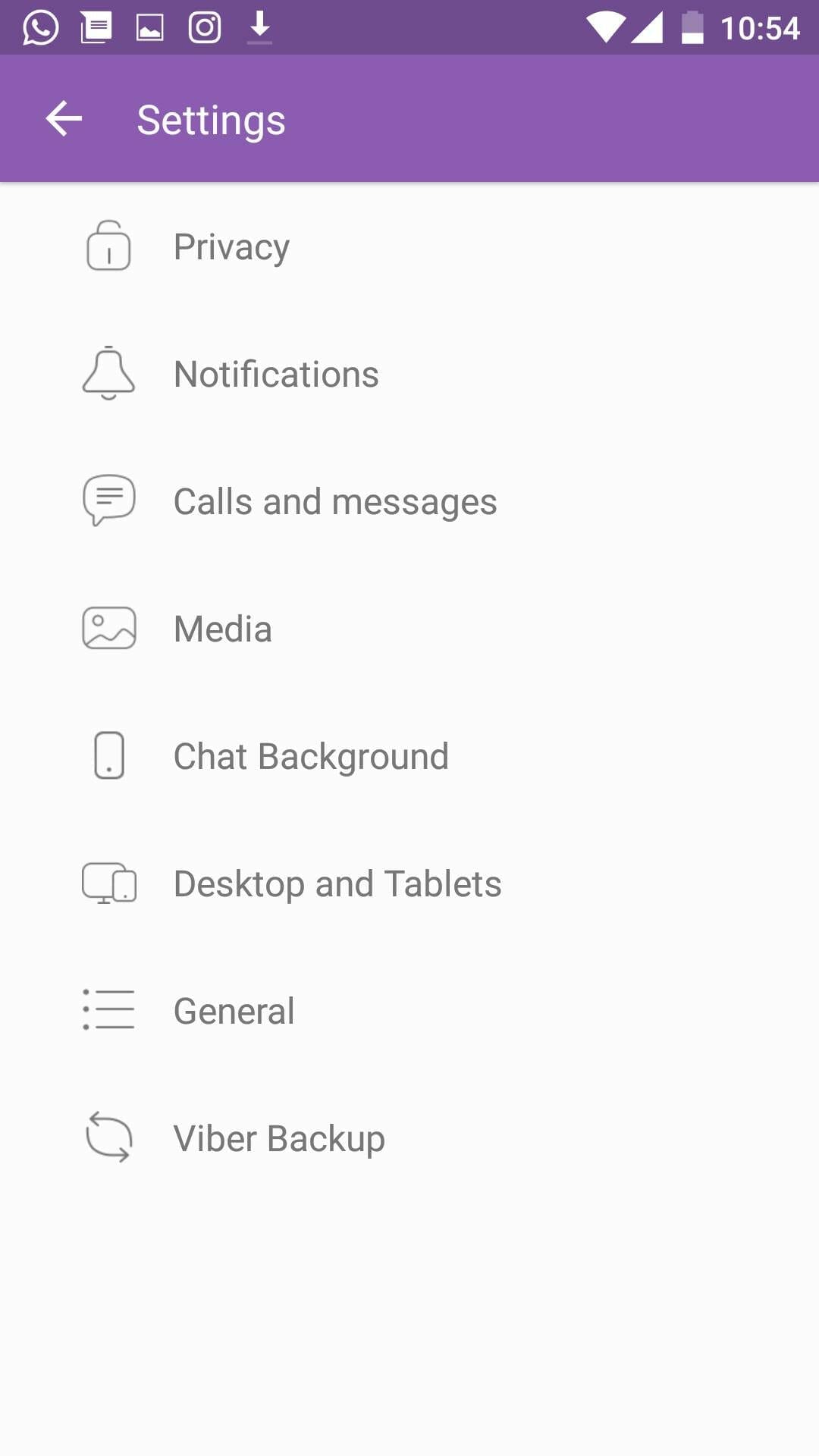The image depicts an app's settings page. At the very top, the status bar displays various indicators including battery percentage, current time, and Wi-Fi signal strength, all against a purple background. A white back arrow and the word "Settings" are also visible in this top section.

Below the header, the page transitions to a white background with gray text and matching gray icons for each settings category. The first setting is labeled "Privacy" and is represented by a lock icon. Following that is "Notifications," symbolized by a bell icon. The next setting is "Calls and Messages," illustrated with a text bubble containing a few lines. "Media" comes next, accompanied by an icon depicting a mountain and a sun.

Continuing down the page, "Chat Background" is indicated by a smartphone icon. Then, there is a "Desktop and Tablets" section, marked by an icon showing both a desktop computer and a tablet. The "General" setting follows, represented by an icon of three lines forming a checklist. The final setting is "Fiber Backup," depicted with two rotating arrows.

Overall, the interface is designed with clear, straightforward icons and text, facilitating easy navigation and user interaction.